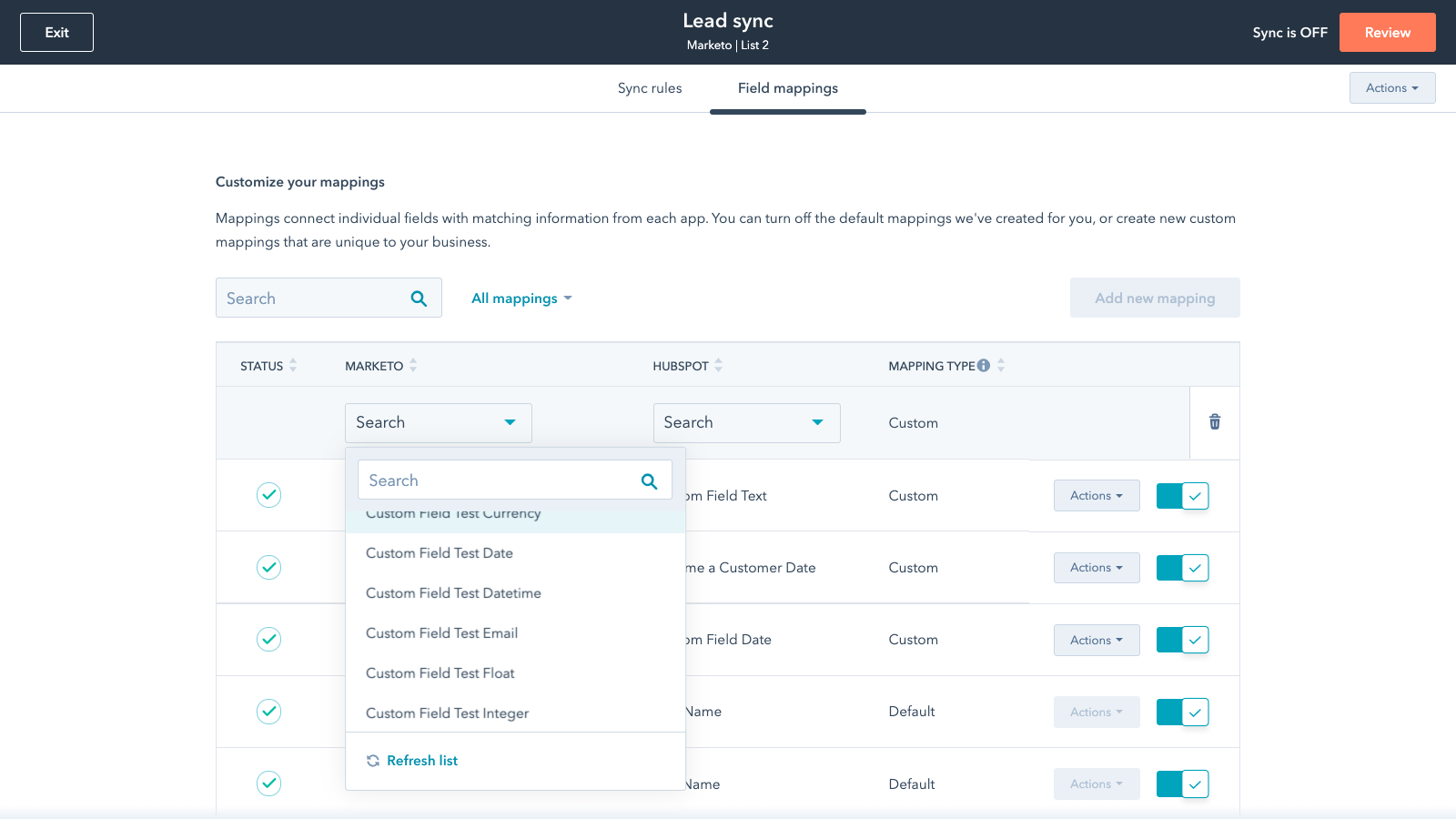**Caption:**

This image depicts the *Load Sync* interface, prominently titled "Load Sync" at the top. On the left side of the screen, there is an "Exit" button, while the right side features a message indicating "Sync is Off" and a "Review" button. The central part of the interface shows "Sync Rules and Field Mappings," guiding users to customize their mappings. It explains that mappings connect individual fields with corresponding information from each app, allowing users to turn off default mappings or create custom mappings unique to their business needs. At the bottom of the screen, a search bar labeled "All Mappings" is visible. In the main section, a table is presented with various columns: "Status" (where all entries are checked), "Marketo," "Search," "HubSpot," and "Mapping Type." This comprehensive layout provides an overview of the syncing options and customization capabilities available to the user.